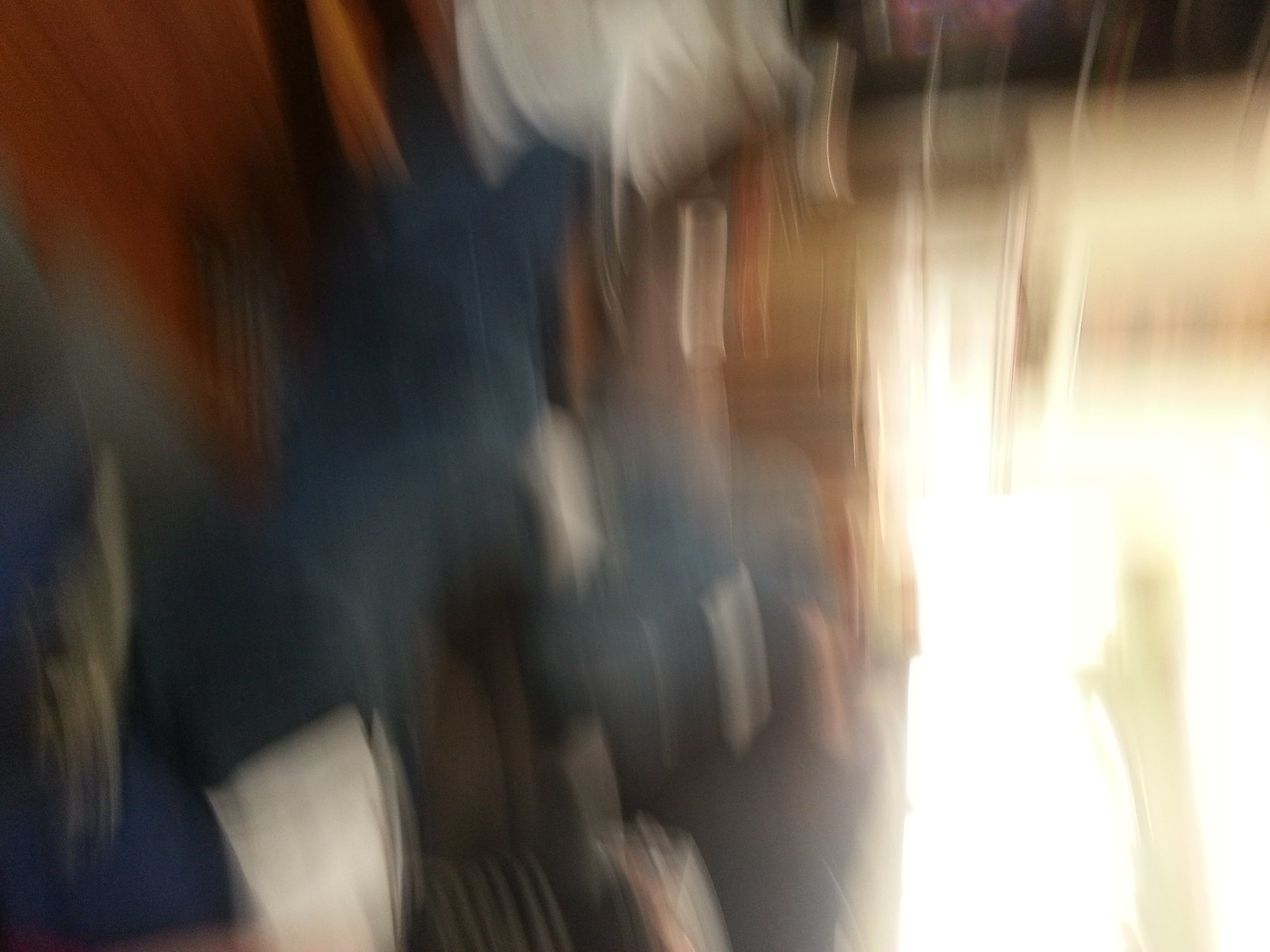The photograph appears to have been taken indoors, capturing a very blurry scene with vertical streaks suggesting the camera was moved downward during the exposure. On the right side of the image, there's a very bright, overexposed area of sunlight, likely coming from a window or a skylight, illuminating portions of the scene. The left side of the image features various colors and objects that are difficult to identify due to the blurriness. There are light blue and dark blue tones, some of which might be pillows or other items, and a red area that could be part of a wall. The background shows what looks like a floor and possibly stairs. In the foreground, on the left, there are several indeterminate objects piled up, with one item resembling a garden hose reel wrapped around a cylindrical holder. The overall base color observed in the image is brown, likely indicating wood surfaces on the wall or floor. The photograph suggests an indoor storage area or a cluttered space, with significant light shining through an opening on the right side, casting a bright shine across the scene.